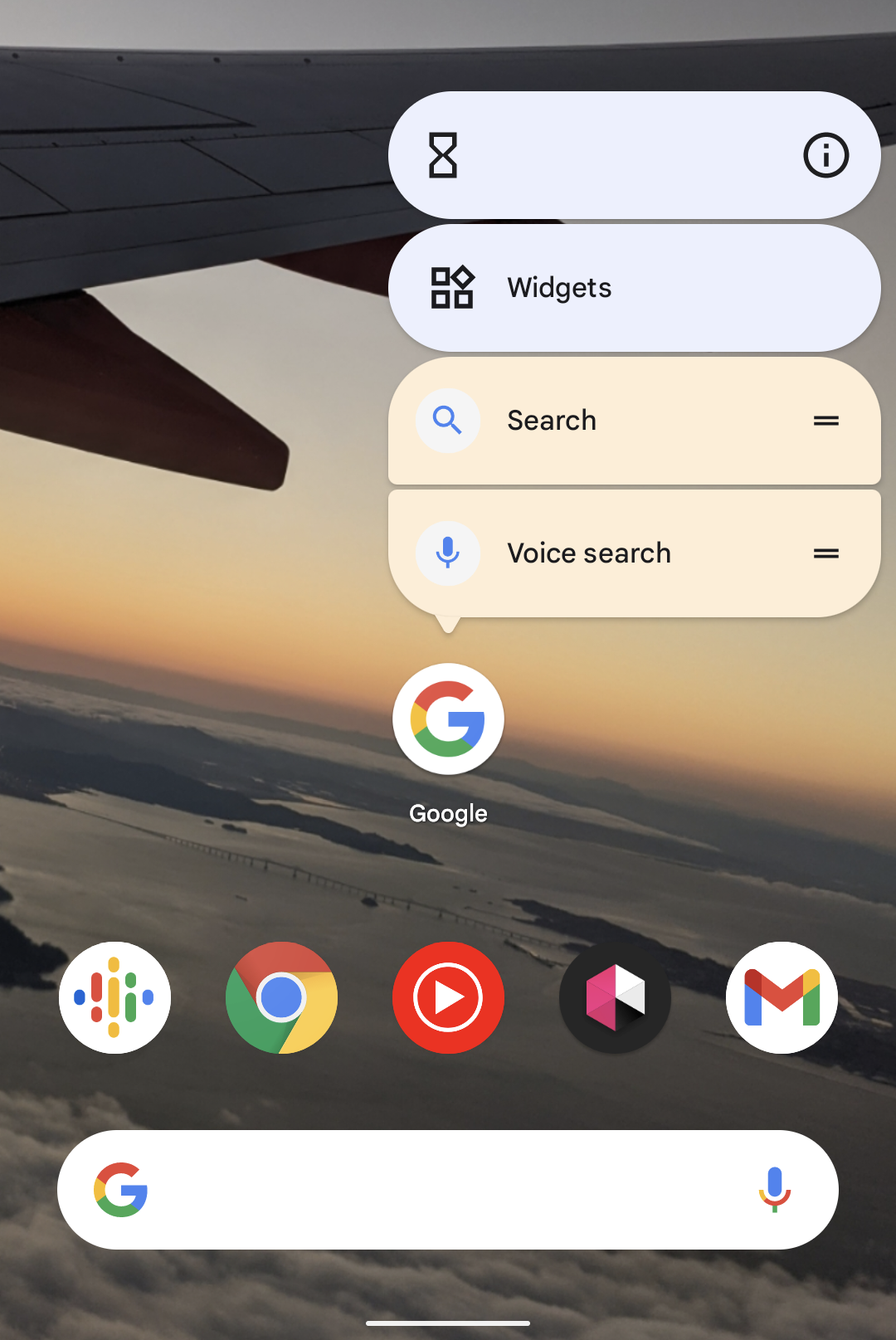The Android home screen features a serene background image captured from a commercial airliner in mid-flight. The vantage point offers a view from a side window, looking out over expansive clouds below. Beyond the clouds, a body of water can be observed, potentially an ocean or a large inland lake, with scattered landmasses dotting the horizon. A distant bridge is barely visible amid the far-reaching landscape. The right wing of the plane is prominently displayed in the foreground, while the sun, already set below the horizon, casts a remaining orange glow across the sky. 

On the screen itself, various app icons are arranged, predominantly those associated with Google. These include the Google app, Chrome, YouTube, and Gmail. A long press on the Google app has revealed context options such as Widgets, Search, and Voice Search. At the bottom of the Google app, a search bar is present along with a microphone icon for voice input. The overall layout of the home screen is minimalistic, with ample empty space giving it an uncluttered and airy feel.